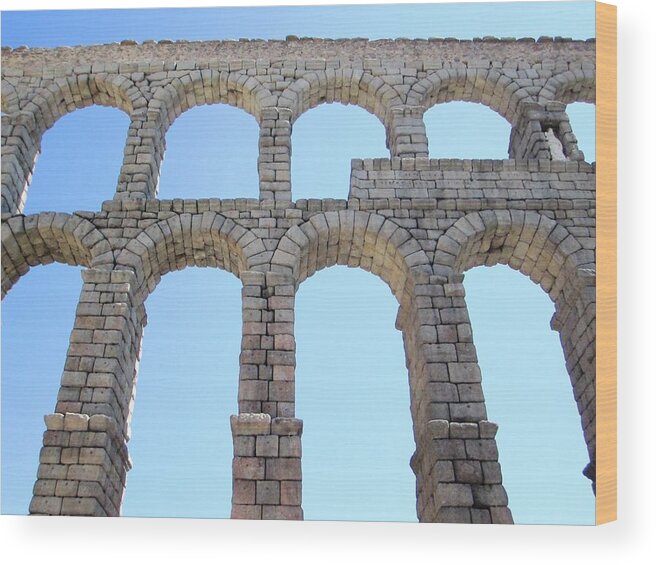The image captures the ruins of an ancient stone structure, possibly reminiscent of Roman architecture such as an aqueduct or viaduct. The perspective is from the ground, looking up at the imposing edifice. The structure is composed of two levels of arches, the lower level featuring four long, narrow arches, while the upper level mirrors the same number of arches but at half the length. The grey stonework, evoking a bygone era, stands against a clear blue sky, with sunlight casting distinct shadows across the weathered surfaces. The edifice appears partially intact, with some sections missing, suggesting it was once part of a larger, grand building, now reduced to its skeletal remains. The viewer's gaze is drawn through the arches, framing the sky, hinting at the grandeur of a now-demolished historical landmark.